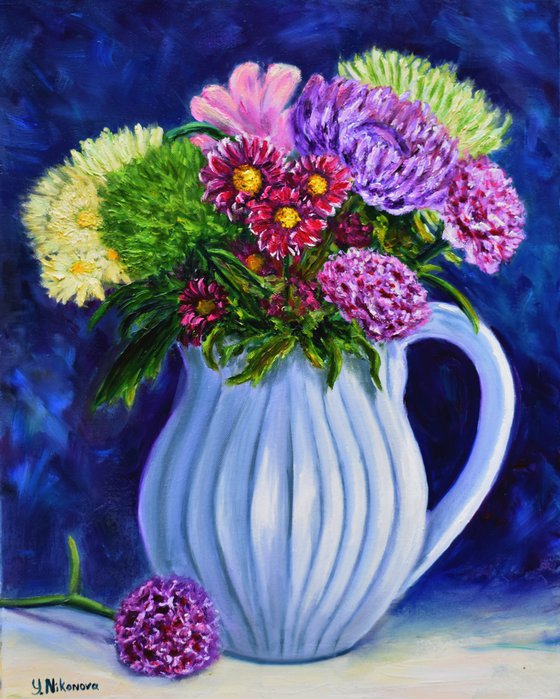This image is a vibrant and richly detailed painting showcasing a tall, round, coruscated vase, which is predominantly white with blue contours and ridges, and featuring a large white handle on the side. The vase holds an abundant and varied bouquet of flowers in vibrant colors, including bright greens, pinks, purples, reds, and yellows, with some flowers even exceeding the height of the vase. The bouquet is complemented by dramatic and vividly pigmented colors, creating dynamic visual interest. At the base of the vase, there is a loose blue and a pink-purple carnation, adding further layers of detail. The background of the painting features a deep, churning blue-purple mass with lighter highlights, enhancing the sense of depth and intensity. The bottom left corner of the painting bears the artist's signature, "Y. Nikonova," in black, indicating the creator's identity. Overall, the painting exudes a sense of professional artistry, with careful attention to color, texture, and composition, resulting in a masterfully crafted depiction of floral elegance.